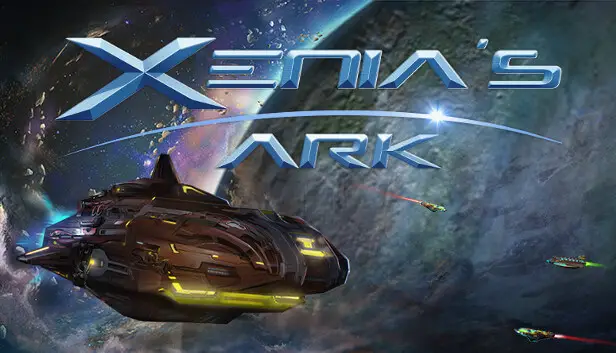The image appears to be a still from a video game set in outer space. Dominating the background, the scene showcases a cosmic expanse with deep shades of purple, blues, grays, and blacks, giving an ethereal sky-like impression. A large, rounded shape on the right-hand side suggests the presence of a planet enveloped in dark blue and gray hues.

Prominently across the top-middle section of the image, the title "Xenia's Ark" is displayed in a futuristic blue font. The letters feature a sleek, modern design, with elements that appear almost 3D and slightly disconnected—emphasizing the advanced theme. Between "Xenia's" and "Ark," a blue line arches in a rainbow-like curve.

In the lower left corner of the image, there is a futuristic spacecraft, colored in shades of light brown with striking yellow lights. This vehicle resembles a space-traveling car and is positioned as if it is moving forward. On the bottom right, three smaller, equally advanced spacecraft emit red and green laser-like lights, adding a sense of dynamic action to the scene. The combination of these elements creates an awe-inspiring depiction of a futuristic outer space adventure.